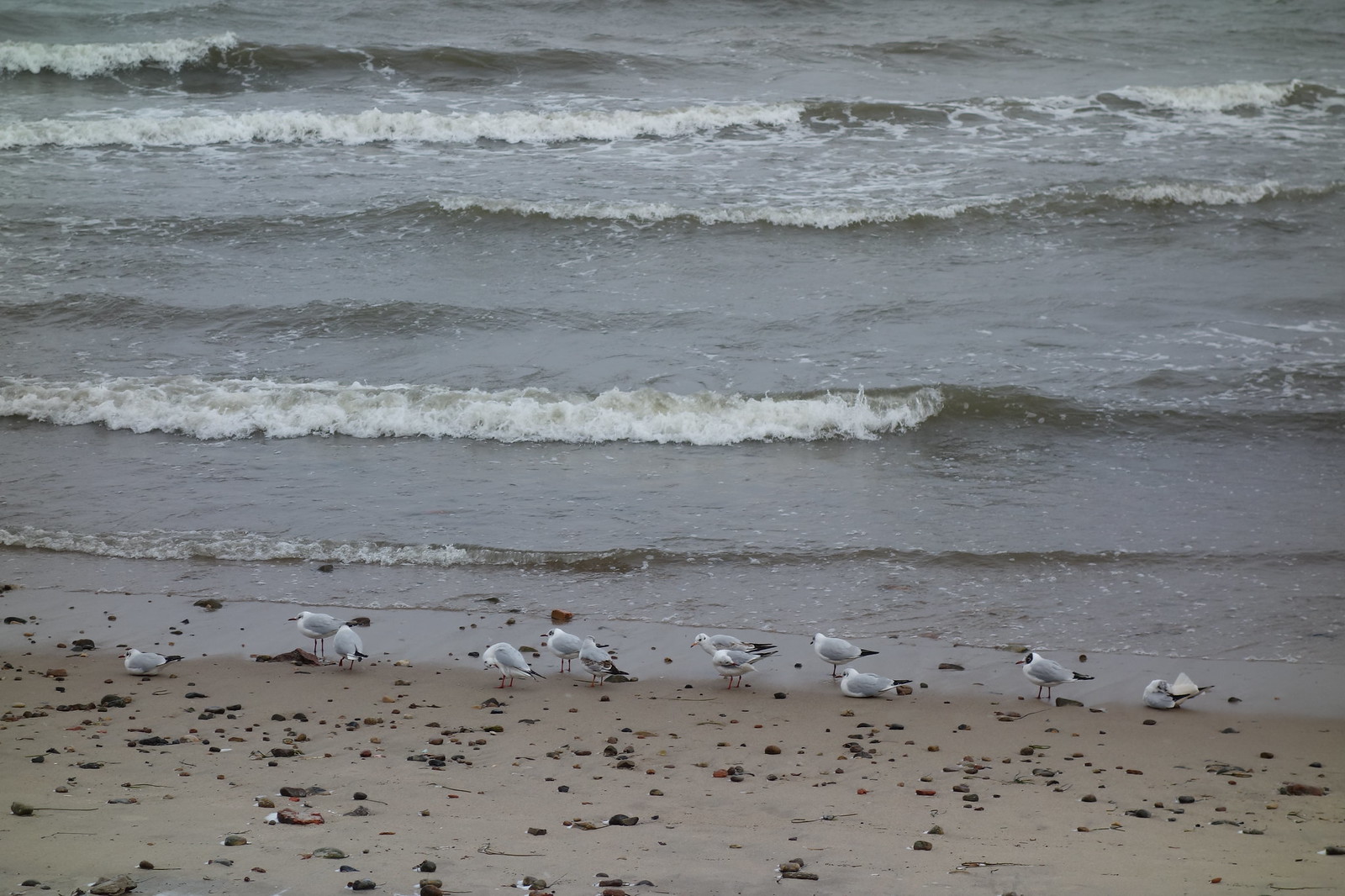This photograph captures a serene beach scene on an overcast day, characterized by its gray, cloudy skies and a similarly gray, plain expanse of water with small whitecaps gently rippling towards the shore. Along the wet, debris-strewn sand close to the water's edge, a group of approximately ten seagulls with distinctive grey backs, white heads, black tail feathers, and small beaks are positioned. Most of the birds are standing still, with one lying on the ground, potentially probing the sand for small shellfish. The composition highlights the natural details of the shoreline, including the textured sand dotted with stones and holes, contributing to the scene's overall tranquil and somewhat somber atmosphere.